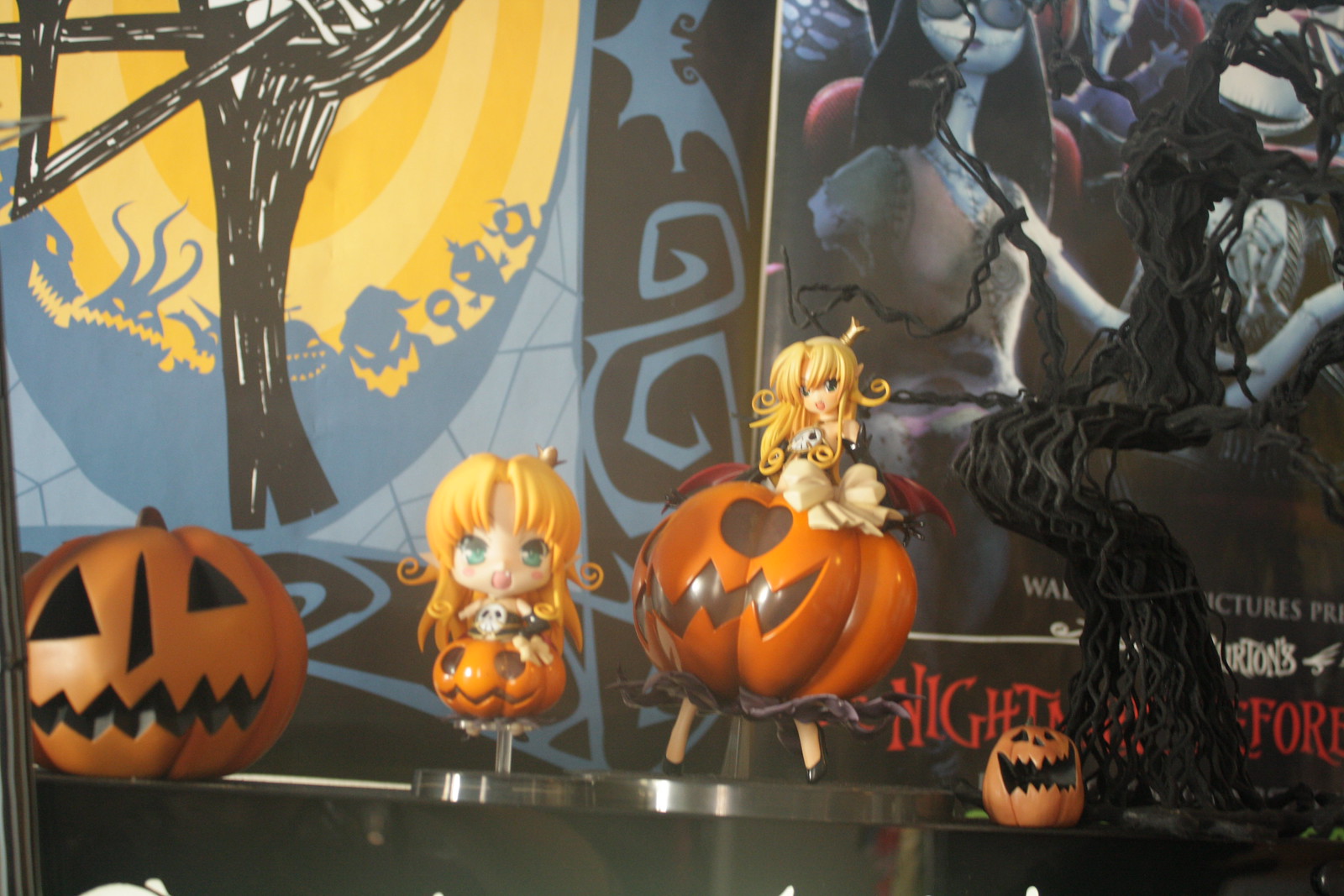The photograph captures an elaborate Halloween scene featuring a detailed arrangement of figurines and decorations. On the right side stands a spooky tree model composed of twisted vines, accompanied by a small jack-o'-lantern at its base. On the far left is a larger jack-o'-lantern with a more closed mouth. Between these two pumpkins stands an anime character dressed in a festive jack-o'-lantern outfit. Two versions of the character are depicted: one in chibi style with a large head and huge, expressive eyes, attached to a clear pole, and the other in black high heels, wearing the pumpkin as part of her attire along with a skull tube top. This character features distinctive blonde curly hair. The background includes an array of Halloween-themed drawings and decorations, including eerie images from "The Nightmare Before Christmas" and a poster for the film. Elements like a haunted black-draped tree, plastic jack-o'-lanterns, and two blonde dolls holding skeletal figures make the scene rich in Halloween spirit and detail.